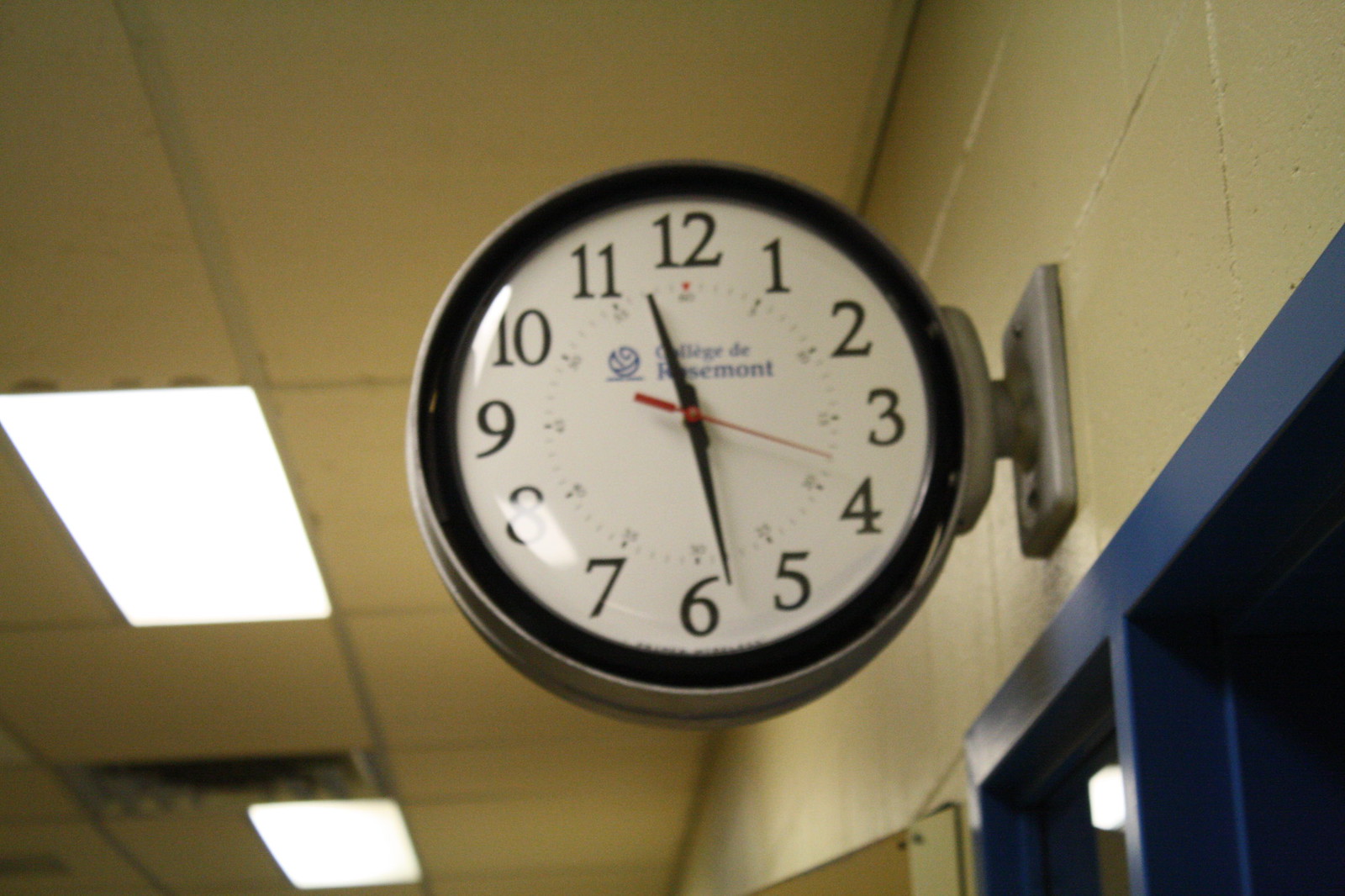This detailed photograph captures a close-up of a slightly older, double-sided wall clock, likely from the 80s or 90s, mounted in a hallway, which suggests a school-like environment or possibly a hospital or business building. The clock face displays the time as 11:28, with black hands and a second hand positioned between the 3 and 4. The clock features black numbers on a white background, encased by a black bezel, and a grey mount attaching it to the wall. Above the door frame with blue metal trim, the clock bears the name "College de Rosemont" or "College de Fairmont" along with a small logo. The setting includes cinderblock walls painted an eggshell or pale yellow hue, influenced by the fluorescent lighting visible in the ceiling tiles above. The ceiling appears off-white due to lighting but might be yellowish. This image gives off a nostalgic vibe, depicting a quiet hallway with a standard institutional ambiance.